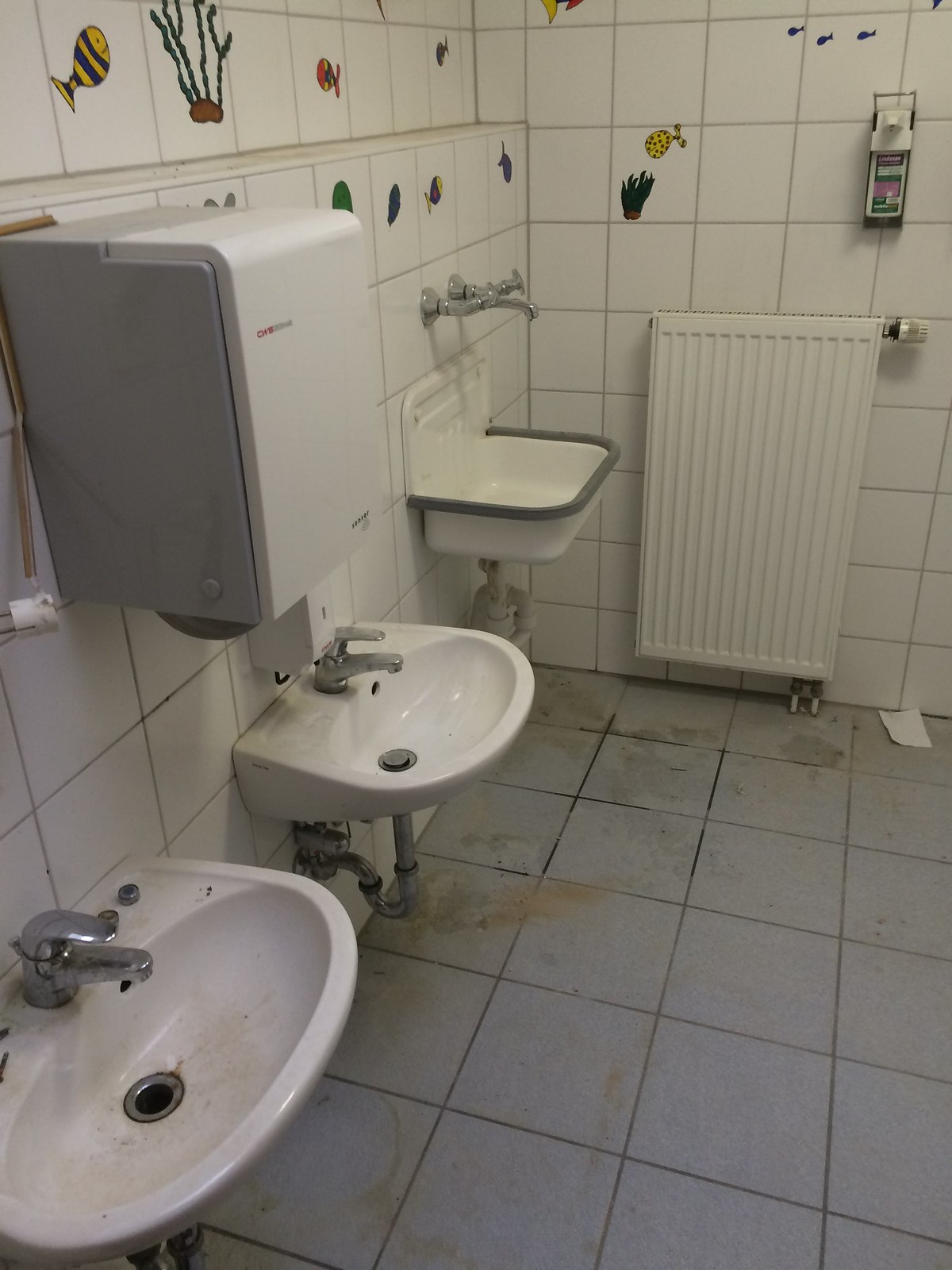This image captures a rather grimy corner of a children's public bathroom, likely in an elementary school. On the left side, lined up against a wall of large white tiles adorned with stickers of fish and underwater plants, are three white sinks. The two sinks closest to the foreground are oval-shaped, low to the ground, and feature mixer taps. Above and between them, there's a white paper towel dispenser with gray sides and a soap dispenser mounted on the wall. The third sink, farther back and distinct in style, has a deeper basin with separate hot and cold water taps, appearing more utilitarian. The floor of this bathroom is covered in gray, non-slip tiles, which are notably stained and dirty. Opposite the sinks, against the back wall, stands a white radiator partially enclosed by a cover. The entire scene is dominated by a sense of neglect, with visible rust, water spots, and brown marks in the sinks, adding to the overall unkempt appearance.